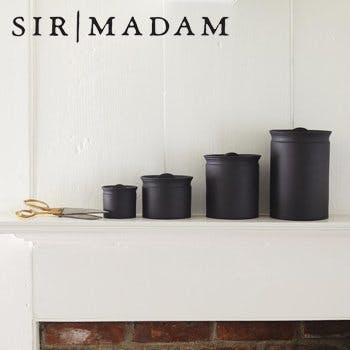This image features a set of four black canisters of varying heights arranged on a pristine white mantel, which appears to be above an old red brick fireplace with gray mortar. The canisters are cylindrical in shape with black lids, each topped with a small black handle dot. From left to right, they increase in size, with the smallest positioned next to a pair of elegant scissors boasting gold handles and silver blades. The white mantel contrasts sharply with the surrounding white walls and the red bricks peeking out from below. In the top left corner of the image, the text "Sir / Madam" is displayed with a black line dividing the words. The overall composition suggests a carefully curated and seldom-used fireplace area.